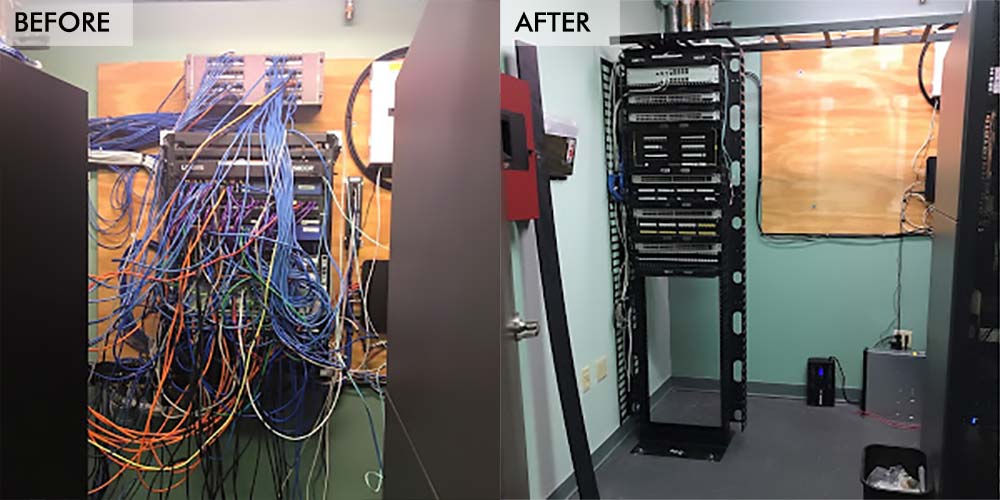The image consists of two side-by-side photos labeled "before" on the left and "after" on the right, showing a dramatic transformation of a server room. In the "before" shot, the room is cluttered with a chaotic tangle of blue, orange, white, black, and red cables sprawling in every direction. Panels and cords create a disorderly mess against a wooden backdrop, with cords plugged into various devices. The "after" image reveals a significantly tidier setup, where most of the cords have been eliminated, and the server equipment appears organized in a sleek, black metallic frame with only a couple of cables visible. The setting emphasizes a clean and efficient workspace, indicating that some professional organization or server cleanup took place, though no specific information about who performed the work is provided. The overall impression is a dramatic improvement in organization and tidiness in the server room.